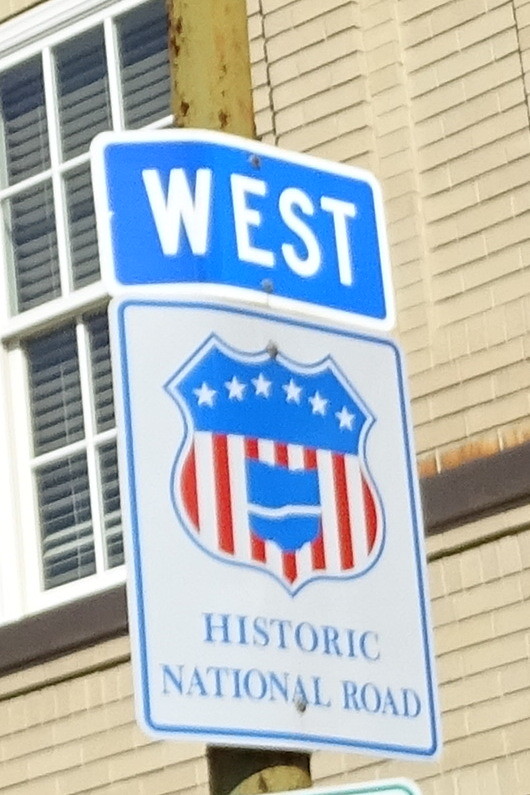The image features a street sign indicating "West" on the Historic National Road. The sign is adorned with white lettering, red accents, and six stars, resembling a barbershop logo. It is attached to a metal street pole. In the background, there is a large window set in beige-colored brick, suggesting the façade of a residential building. Additionally, a brown utility pole is visible nearby. Below the main sign, a partial glimpse of a secondary sign can be seen, hinting at a busy street location. This sign serves to denote the historical significance of the road it marks.